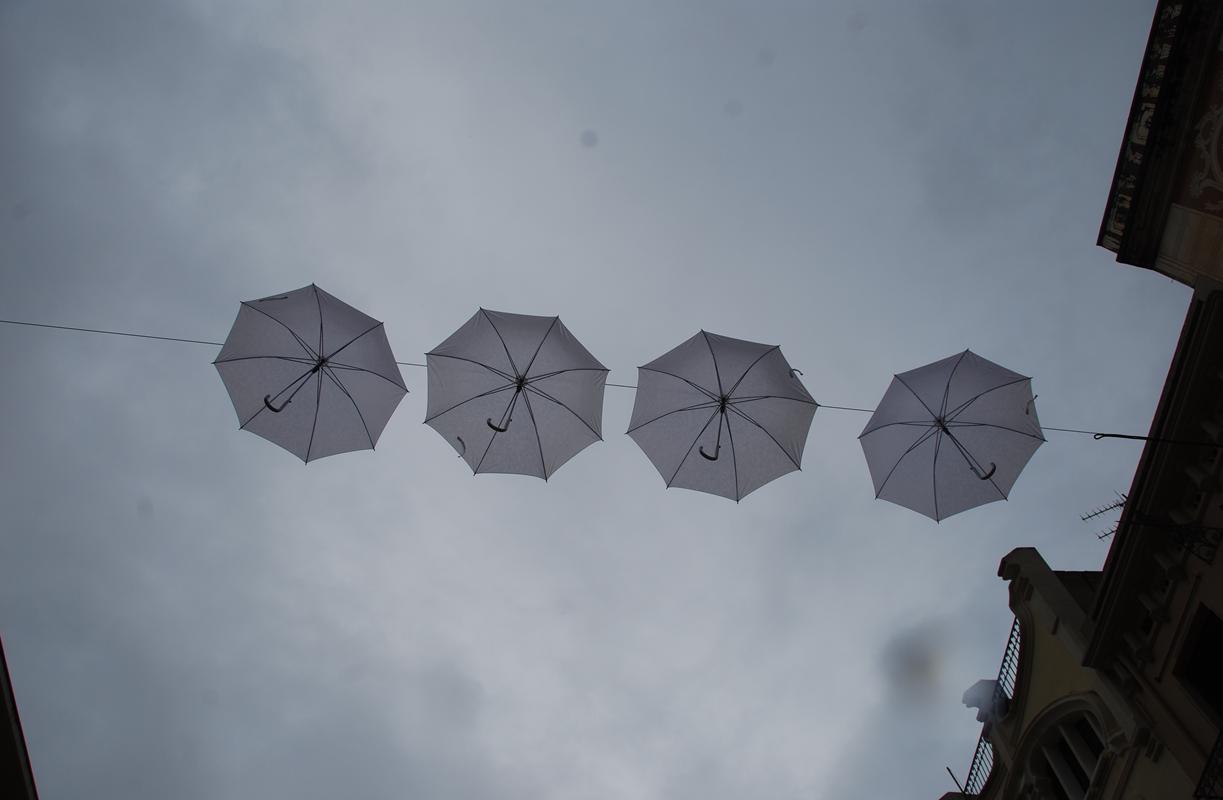In this color photo, you are positioned as if standing on the ground and looking up at a sky that is blue with various shades of gray, suggesting a somewhat gloomy day with patches of clouds. Across the sky from left to right stretches a thin wire or power line, upon which hang four white umbrellas, their handles resembling candy canes pointing in different directions. These umbrellas are spaced evenly along the line and, due to their upside-down positioning, evoke the image of floating jellyfish.

To the right side of the frame, you see the top of a light yellowish-brown building with a railing at the top and three windows beneath it. The left side of the image offers a glimpse of another building's roof, though the full structure is cut off by the edge of the picture. The entire scene feels artistically composed, capturing a sense of dreariness and calm under a potentially rainy sky.